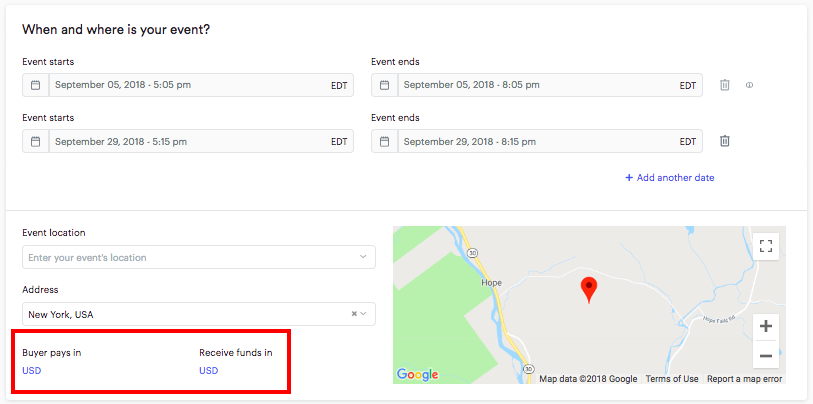The image displays a user interface for event scheduling. It features a white rectangle with a gray border. At the top left, bold black letters ask, "When and where is your event?" Beneath this, in smaller letters, it states, "Event starts." Below this text is a light gray rectangle containing a calendar icon on the left side, a section in the middle to change the date and time, and an "Edit" button on the right side. There are four such sections in the image.

The first "Event starts" box indicates "September 05, 2018, 5:05 PM," and the second one shows "September 29, 2018, 5:15 PM."

To the right, there are two boxes labeled "Event ends." The first indicates "September 05, 2018, 8:05 PM," and the second displays "September 29, 2018, 8:15 PM."

At the bottom right corner, there is an image of a Google Maps interface.